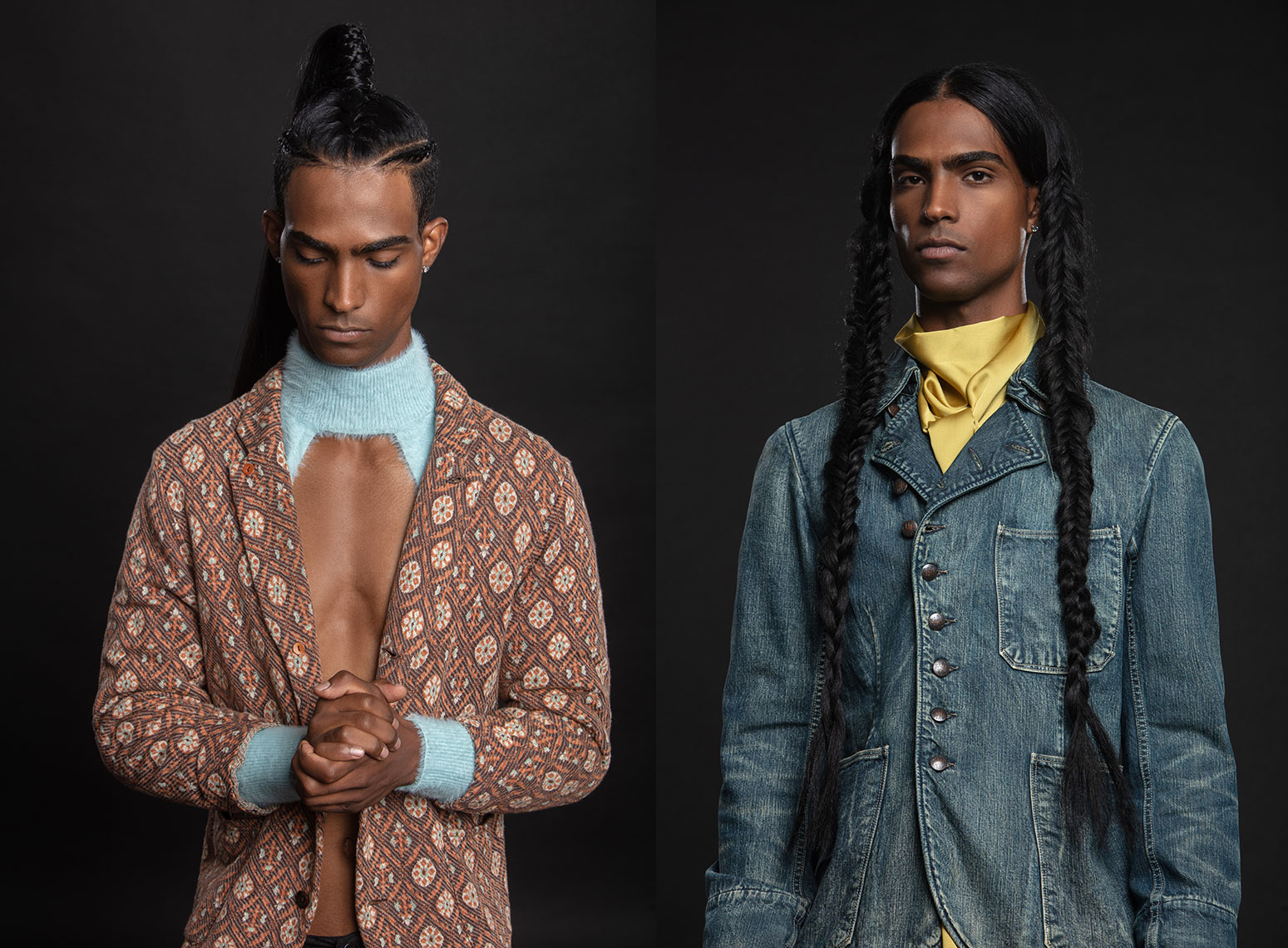The image depicts two men, possibly of Native American or African heritage, both with dark skin and black hair styled distinctly. The man on the right wears his long hair in two braids reaching his waist. He dons a buttoned-up blue jean jacket with silver buttons and a yellow, silky undershirt. An earring is visible in his left ear, and he gazes directly at the camera, his hands relaxed by his sides.

In contrast, the man on the left has his hair pulled up with side parts, forming a high ponytail that cascades down his back. He wears a dark brown corduroy jacket adorned with a pattern of whitish circles with brown centers and a blue-collared open shirt, exposing his chest. His head is bowed, eyes fixed on his clasped hands, adding a contemplative touch to his demeanor.

Both men are shown from the waist up, presenting contrasting yet complementary styles that highlight their cultural attire and individual features.